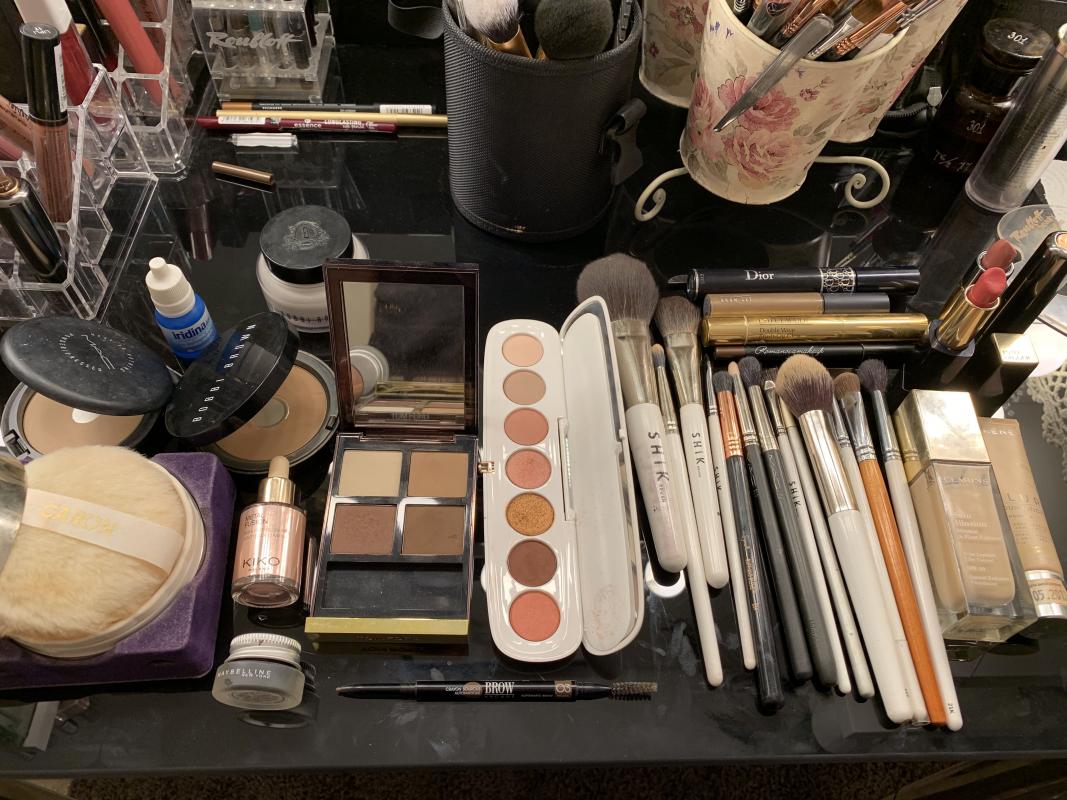The photograph captures a bustling makeup workshop, presumably belonging to a professional makeup artist who works on TV shows or movie sets. The workspace is brimming with an array of makeup tools and products. Foremost among these are numerous makeup brushes—approximately 15 in total—ranging from large, fluffy brushes to smaller, precision brushes, all meticulously organized in cups and pen holders. Various colored makeup palettes are spread open, displaying an impressive spectrum of hues, ready to be applied to enhance the appearance of individuals for the camera. Additionally, an assortment of lipsticks and pencils can be seen, further contributing to the diverse collection of beauty products. There are no visible brand names, emphasizing the focus on the sheer variety and readiness of the tools at hand. The scene embodies the organized chaos typical of a professional makeup environment, dedicated to creating flawless looks for on-screen talent.